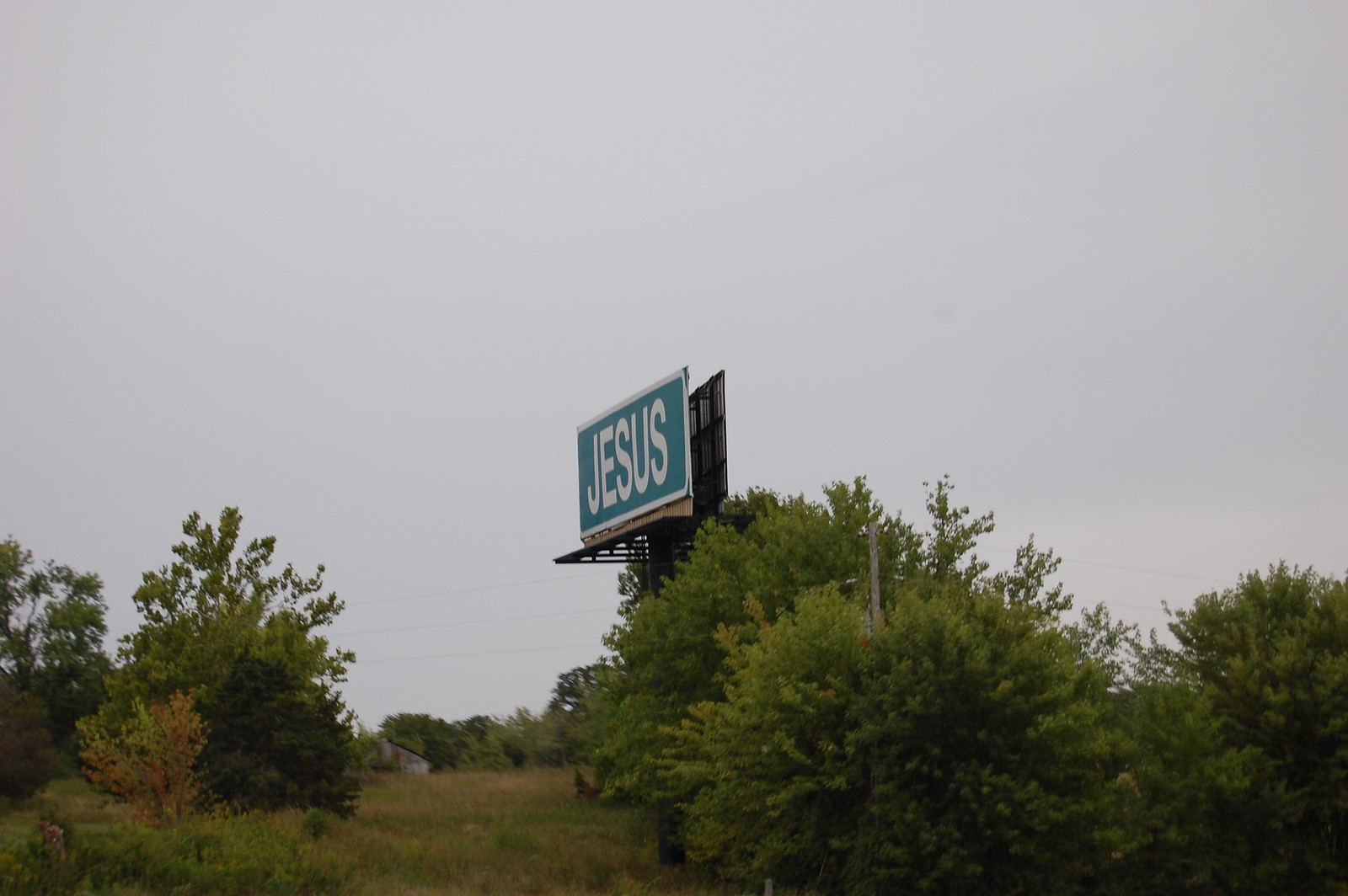In this image, a large green billboard with the word "JESUS" prominently displayed in bold white letters stands out amidst a countryside scene. The sky is overcast, casting a gray hue over the landscape, which features a grassy field dotted with trees. Some of the grass appears slightly brown, hinting at a seasonal transition. Surrounding the billboard, the trees are primarily covered in green leaves, with a few displaying the early signs of color change. The trees also obscure the billboard's stand, integrating it into the natural backdrop. In the distance, a rustic wooden barn—distinct from the typical red barns—can be seen among the trees, which extend across the background. Notably, there are no visible roads in the picture, as the treeline marks the cutoff point of the image. The billboard's message is visible from multiple directions, suggesting there could be duplicate billboards facing opposite ways.